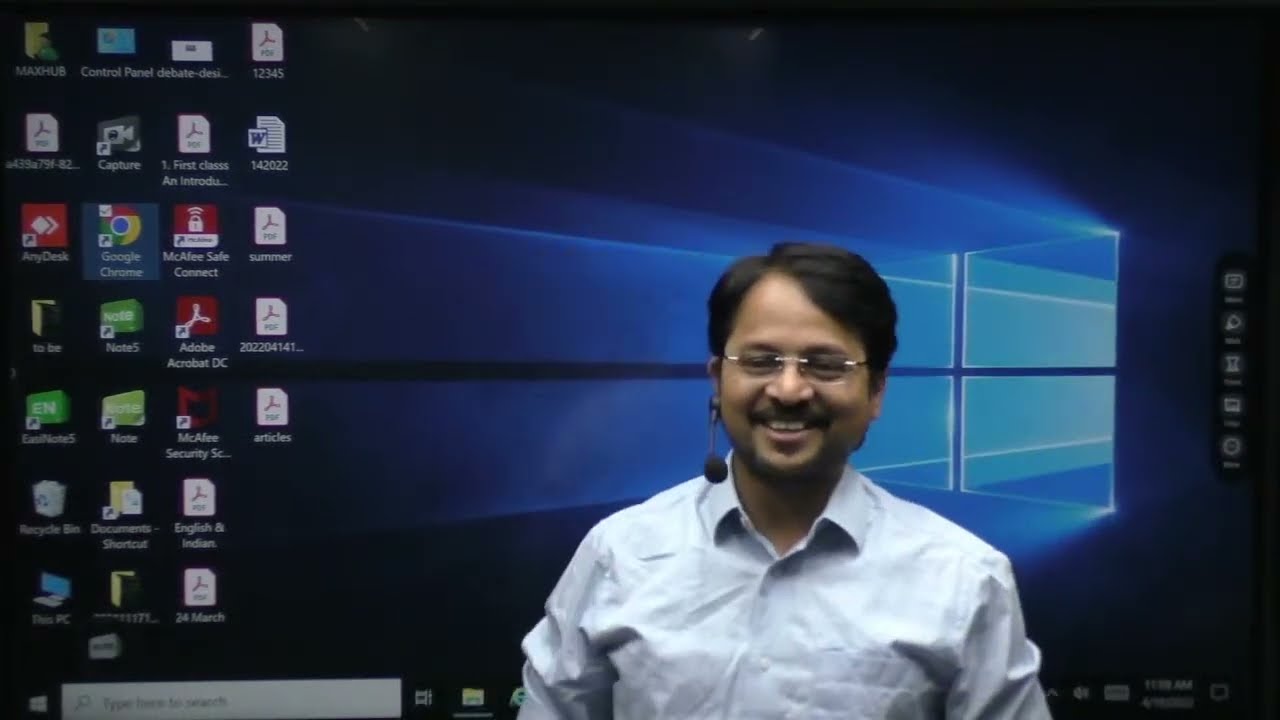A middle-aged Indian gentleman is standing in front of a computer screen background, positioned toward the middle-right side of the image. He is visible from his torso up, wearing a blue button-down formal shirt, glasses, and a headset with a microphone. He has black hair, a mustache, and is smiling warmly at the camera. The screen behind him displays a Windows logo prominently in bright blue, fading into black toward the edges. The left side of the screen is cluttered with several rows of application icons, including recognizable ones like Chrome and Adobe. The arrangement consists of four icons per row, except for the bottom two rows, which have only three icons each. At the bottom-left corner of the screen, there's a white search bar with the gray text "type here to search." The image suggests a virtual meeting or podcast setup, with the man facing forward and engaging directly with his audience.